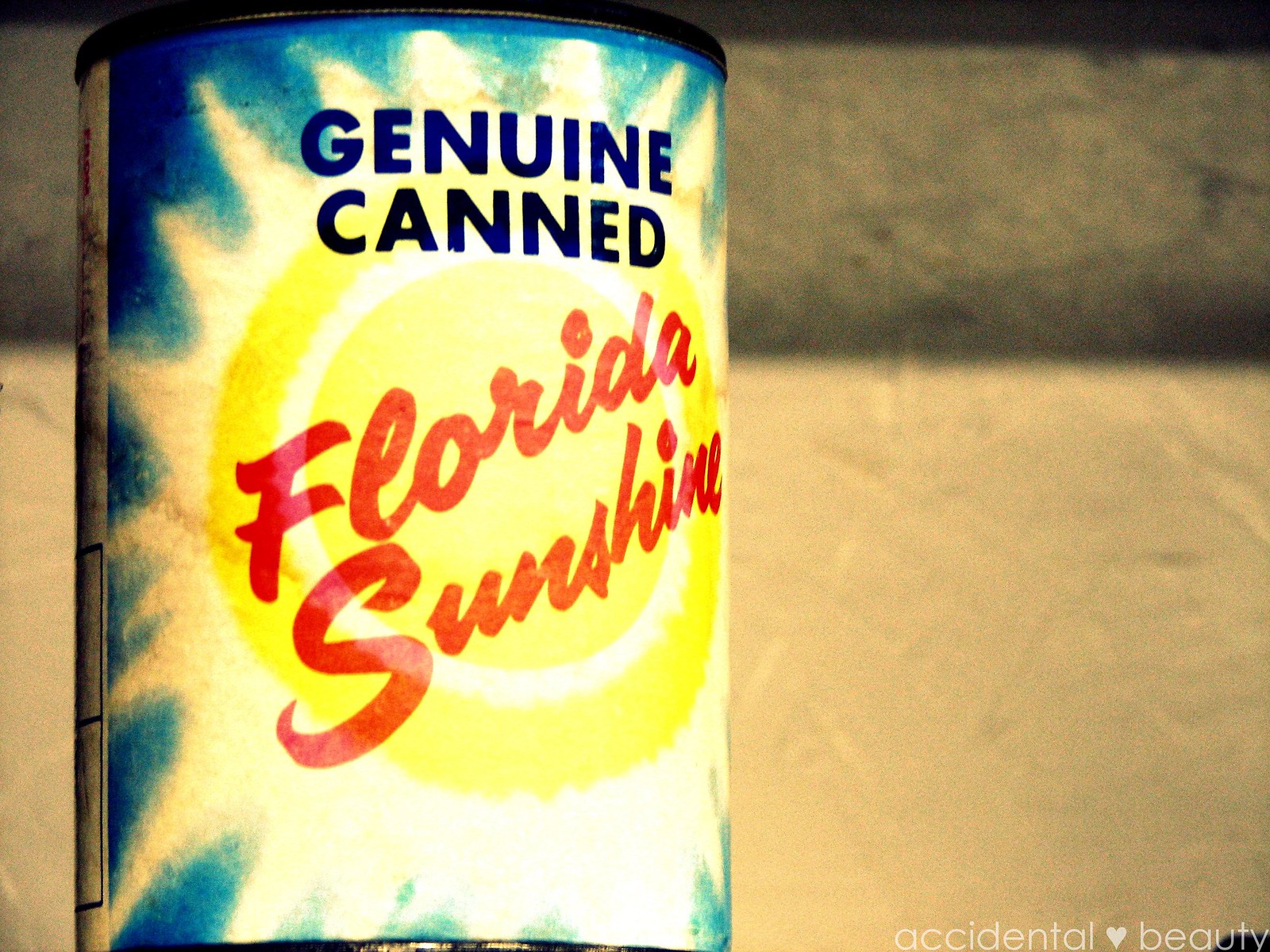This image features a photograph of a novelty item, specifically a can with a blue background and a vibrant yellow sun illustration, emitting radiant rays. The can's top is crowned by the words "Genuine Canned" in dark blue block text and adorned with a red cursive "Florida Sunshine" angled across the sun. The can appears to be sealed with a black plastic lid and sits slightly rusty at the bottom, suggesting it might be an antique or a tourist keepsake from past decades. The background of the image is plain, with a strip of black dividing the upper quarter, which is a darker gray, from the light gray bottom half that resembles sand. Additionally, in the bottom right corner, the phrase "Accidental Beauty" and a white heart are present, possibly as a watermark. Overall, this whimsical piece captures the charm of a bygone era's tourist memorabilia.